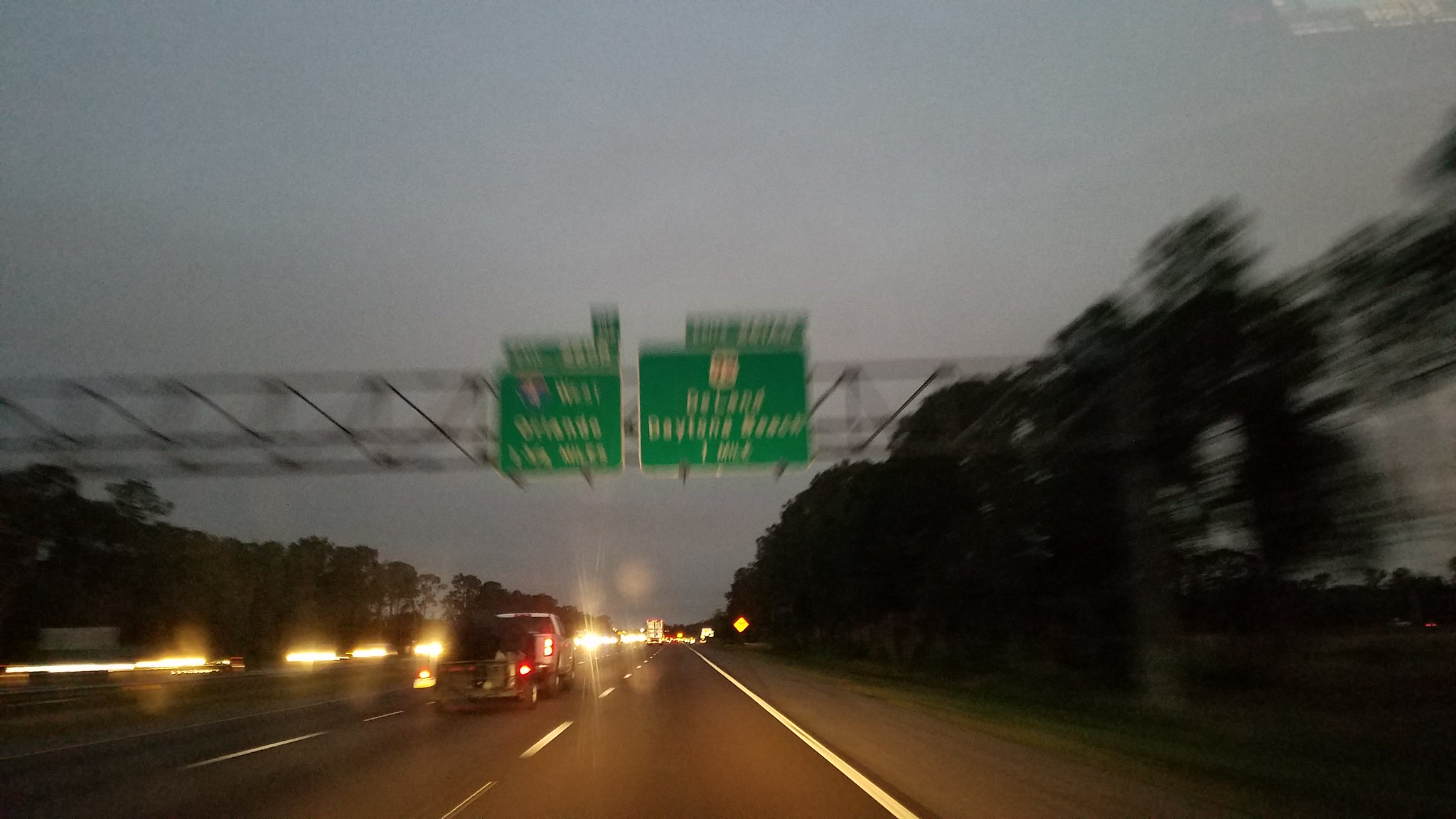This is a vibrant nighttime photograph, seemingly taken through a car windshield while traveling down a freeway. The right edge of the frame lines with the blur of trees, suggesting motion. To the left, headlights beam from the oncoming traffic in the opposite lane, casting a soft glow across the pavement. In the adjacent lane, a truck with a trailer is visible, its red brake lights bright against the dark backdrop. A partially blurred overhead sign stretches across the roadway, the unclear text possibly indicating directions such as "West 5." The overall scene is a compelling mix of illuminated details and shadows, capturing the essence of nighttime travel.